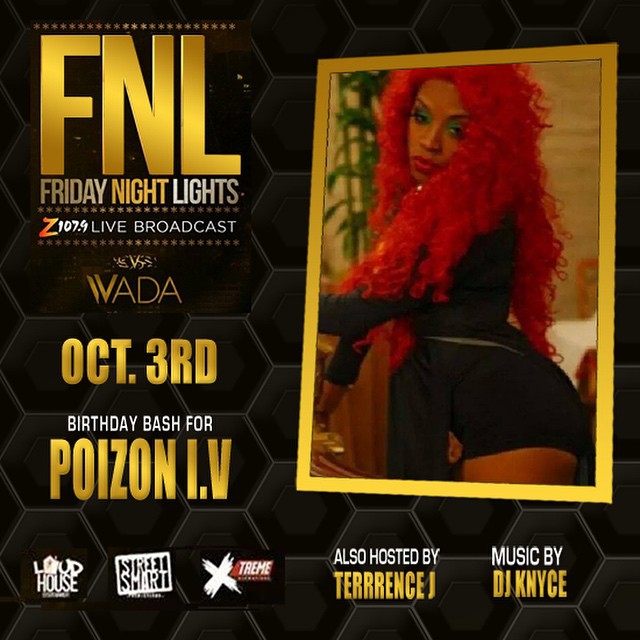This visually striking poster, set against a black background, prominently features the bold golden-yellow text "FNL" in the top left corner, followed by "Friday Night Lights," "Z107.9 Live Broadcast," and "October 3rd Birthday Bash for Poison I.B." (styled in Roman numerals as I.V). Beside this text, within a golden square frame, is a striking photograph of a woman with waist-length, thick, curly or wavy red hair, adorned with red lipstick and green eye shadow. She is wearing a long-sleeved black top that reaches down to her buttocks. The event is also hosted by Terrence J, with music provided by DJ KNYZE. At the bottom, sponsors for the event, such as Loud House and Street Smart Extreme, are listed.